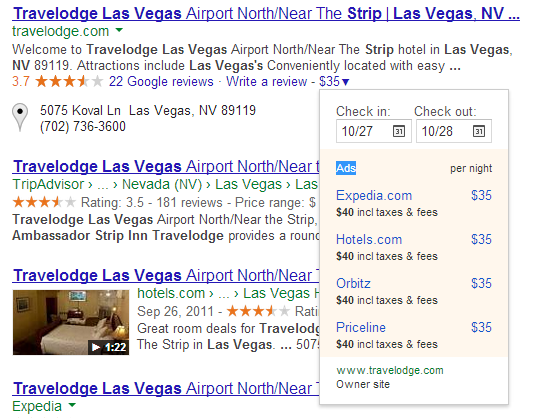This image showcases a Google search results page for "Travelodge Las Vegas Airport North near the Strip, Las Vegas, Nevada." At the very top of the page is the official Travelodge website, Travelodge.com, followed by TripAdvisor and other similar listings. Each result includes standard information about the hotel, with some entries featuring pictures of a bed and an option to watch a video tour of the room, enhancing the appeal by providing a visual preview of the accommodations. The search also displays check-in and check-out dates of October 27 and October 28, respectively, along with pricing information. Multiple booking platforms, including Expedia, Hotels.com, Orbitz, and Priceline, offer rates of $35 per night, which totals approximately $40 when taxes are included. Overall, the page suggests that travelers have several affordable options for staying close to the Strip in Las Vegas.